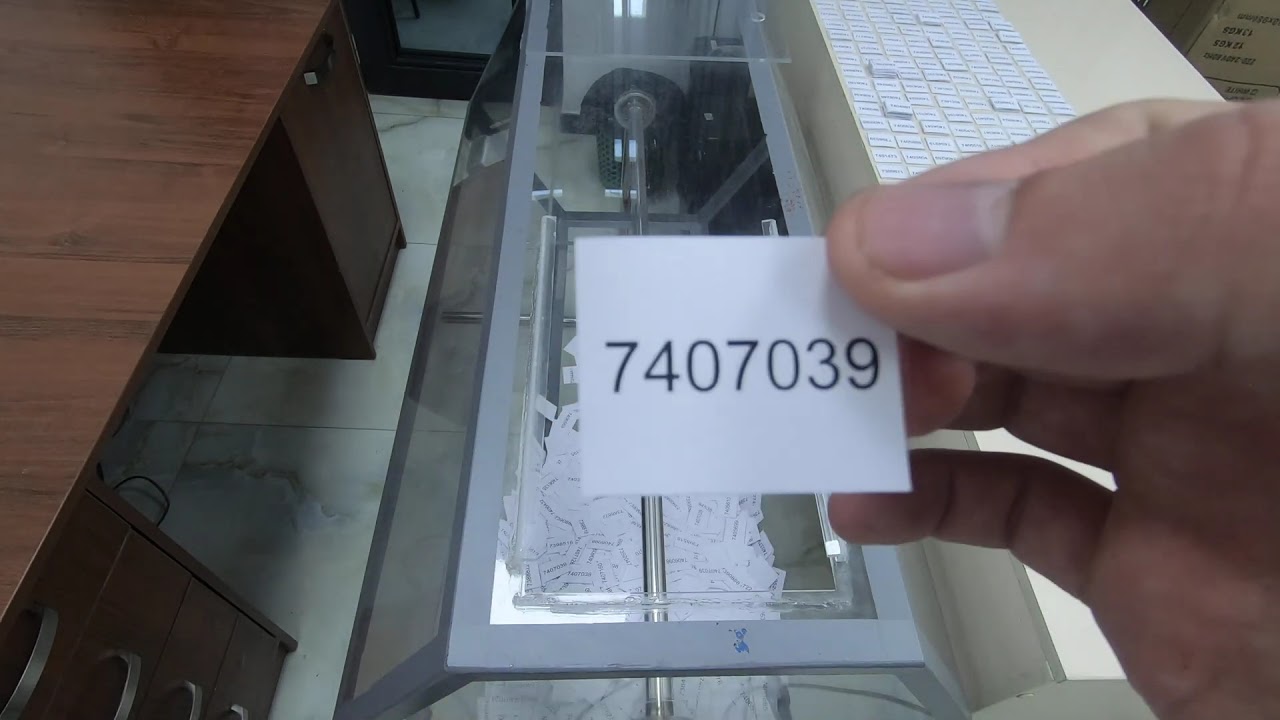The photograph captures a close-up of a white hand clutching a small white square piece of paper prominently displaying the number 7407039. The hand, only partially in view, holds the paper near the right side of the image, centrally positioning the paper itself. Surrounding this central focus, the background reveals a busy, detail-rich scene. To the right, a table strewn with similar small white cutout numbers is evident, alongside a plastic container brimming with these numbered squares. This container reflects light from an overhead source, hinting at a reflective, perhaps glass, surface. On the left side of the image, partially cropped, a dark wooden desk with visible drawer handles adds a contrasting texture. Dominating the central background, a glass contraption—shaped somewhat like a pyramid or coffin and holding multiple paper numbers—features a long, silver spindle running vertically through it, indicating its purpose as a mixing or holding device for the small numbered slips. At the far end of the scene, black machinery is faintly visible, completing the complex and detailed workspace setting.